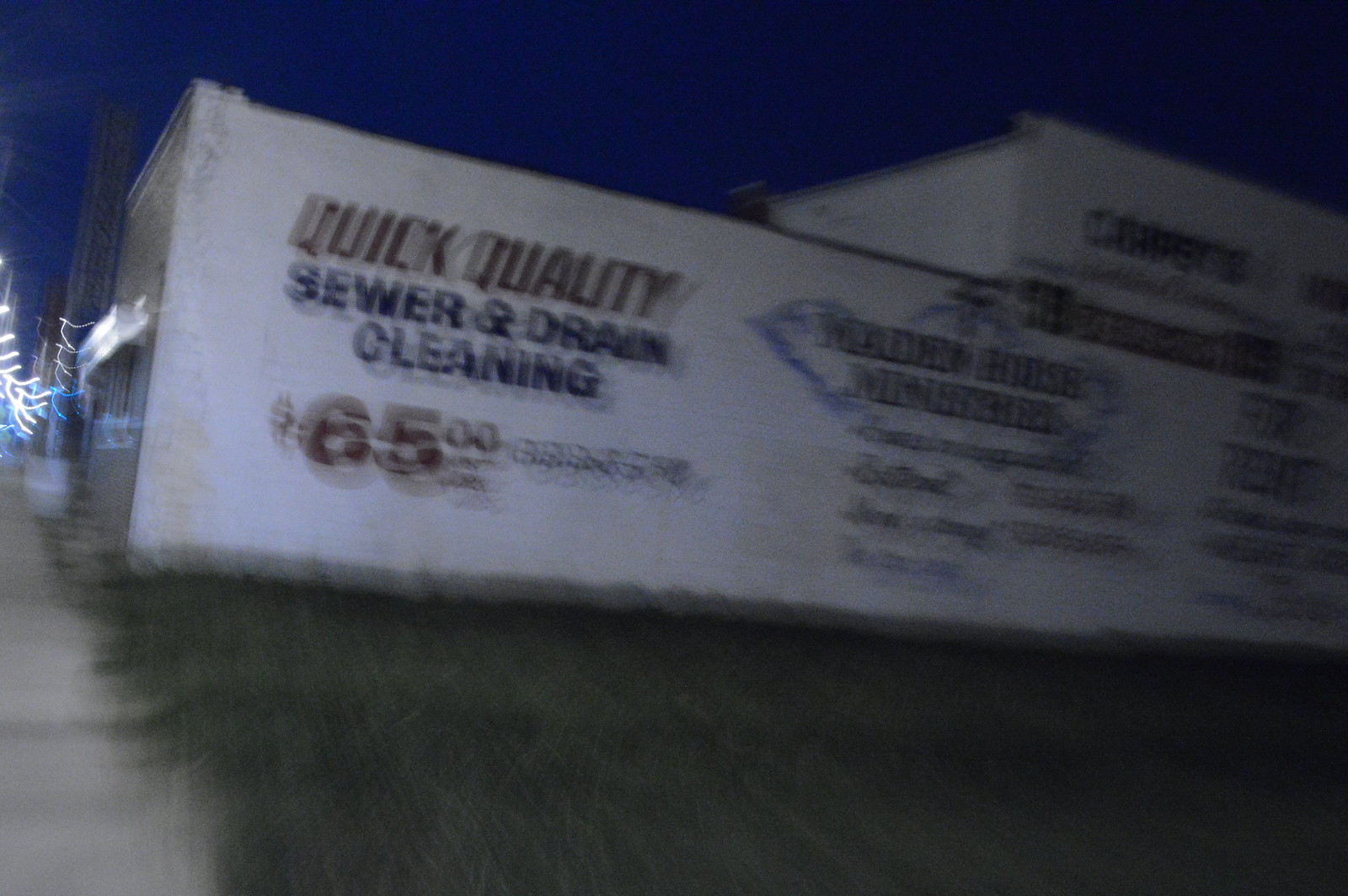This nighttime photograph captures the side of a large, white-painted building adorned with various advertisements. The image, which is notably blurry due to being taken in motion, features vibrant green grass and a light-gray sidewalk running alongside the building. The background reveals a clear yet very dark blue sky. Near the center-left of the photo, dimly illuminated lights create streaks, adding to the mysterious atmosphere.

Prominent on the building is the text "Quick Quality Sewer and Drain Cleaning, $65," with "Quick Quality" and the price written in brown or gold text and "sewer and drain cleaning" in black text. Additional less legible text includes "Madden House Ministries" accompanied by a small black cross, and nearby, another segment that says "Christ" and "for rent." The lower portion of the image is dark, suggesting that the photo captures the scene transitioning from dusk to complete night. The overall composition includes diverse elements such as the sidewalk, grass, and multiple unclear advertisements, all contributing to a complex, multifaceted visual.